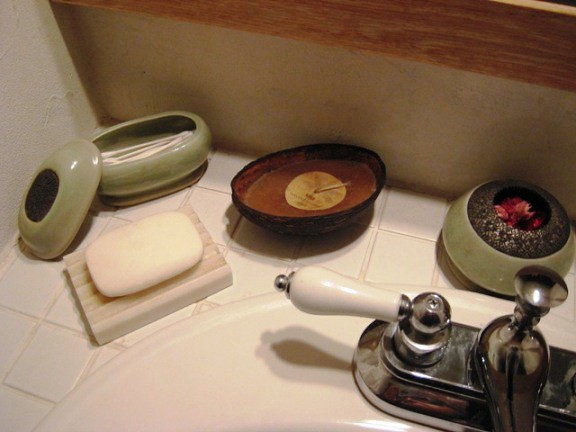The photograph captures the corner of a modest bathroom sink setup, highlighting a few key details. The sink is part of a humble plywood cabinet, paired with a tiled countertop. The image reveals the left side of the faucet, possibly indicating the temperature controls. Alongside the sink, perched on the countertop, is a soap dish meant for holding a bar of soap. Next to this is a quaint ceramic jar with a lid, likely used for storing Q-tips. An interesting candle, almost avocado-shaped, adds a touch of whimsy to the scene. Additionally, a small container, possibly for decorative rocks or possibly housing a tiny cactus plant, brings a hint of nature into this simple, functional bathroom setting.